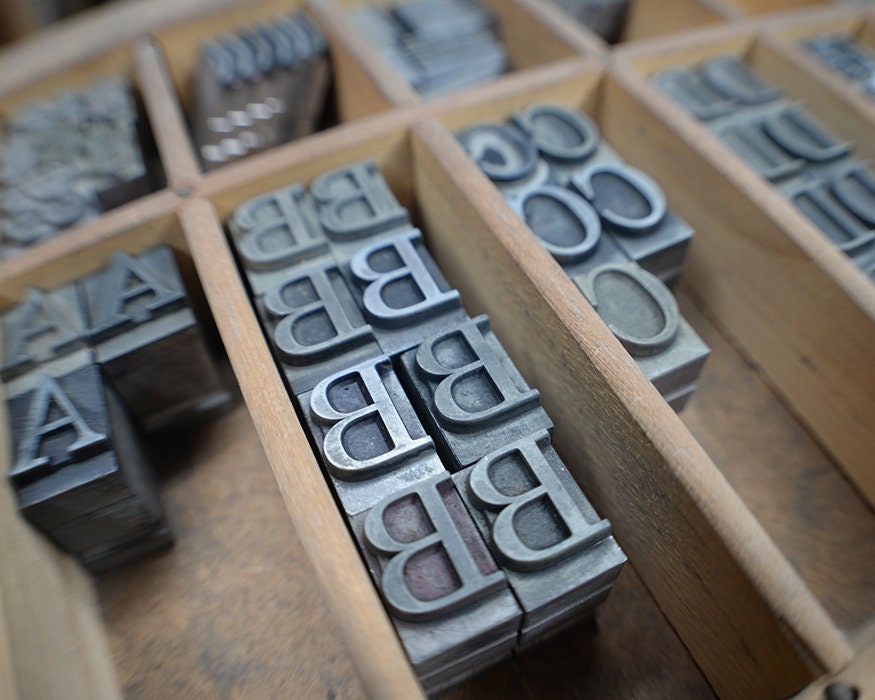The image shows a brown wooden storage box with rectangular compartments divided by wooden panels. Each segment contains stacks of silvery gray metallic cubes with large, capital letters of the English alphabet etched on top. In the bottom left compartment, there is a small stack of letter A blocks. The central focus of the image is on a densely packed section of letter B cubes, arranged in two columns and five rows. To the right, there are several stacks of letter C blocks, organized into three stacks on the left side and two on the right. Following these are the D blocks, though they appear slightly blurred. The image has a shallow depth of field, emphasizing the well-stocked B section amidst the organized array of alphabet stamps. Overall, the scene is distinctly organized within the wooden compartments, highlighting the varying quantities of each letter block.